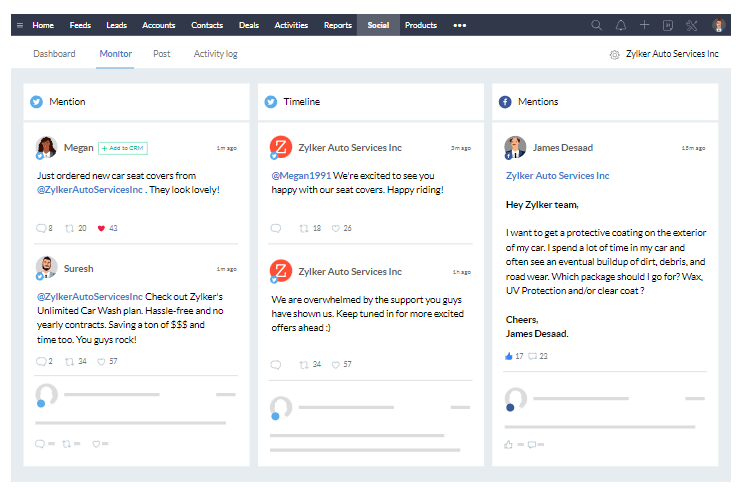The image displays a comprehensive dashboard for a CRM or customer service interface. At the top, a long black navigation bar includes several options with gray backgrounds: Home, Feeds, Leads, Accounts, Contacts, Deals, Activities, Reports, Social, Products, and three small horizontal dots indicating more options. Below this bar, to the left, is the term "Dashboard," and to the right, "Monitor" which is underlined in blue. Further along are "Past" and "Activity Log." 

On the far right, the dashboard is branded with "Zeichler Auto Services Incorporated." The main content area is segmented into different squares representing various interactions. The first section, labeled "Mention," features an image of a person with brown hair wearing a white shirt, resembling an emoji or profile picture. The name "Megan" is displayed, with the text underneath stating, "Just ordered new car seat covers from @Zeichler Auto Services Inc., they look lovely." To the right of this, there's a red circle with a "Z" inside, accompanied by a response: "Megan, we're excited to see you happy with our seat covers! Happy riding!"

Further to the right, another interaction is depicted with a circular image of a man in a suit, identified as James Desad. His message reads, "Hey Zeichler team, I want to get a protective coating on the exterior of my car. Which package should I go for? Cheers, James Desad." A blue thumbs-up icon is next to this message, indicating it has received 17 likes.